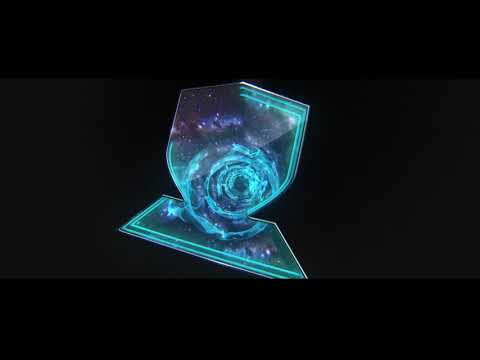This is a highly detailed, computer-generated image resembling a glass or crystal display set against a dark, possibly gaming-related background. The main focus is a complex structure with a flat, trapezoidal base topped by a flat shield-like form. The entire figure appears to be tilted slightly to the right. The base, outlined with blue lights, transitions into the shield, which is highlighted by cyan or light blue borders. At the center of this shield, a swirling vortex or wormhole emanates, featuring concentric circles of vibrant blue and purple lights spiraling into a dark core. This central vortex is surrounded by a backdrop of a purple galaxy or nebula, with additional stars scattered throughout, lending a cosmic ambiance to the scene. Black bars at the top and bottom of the image suggest it might be a screenshot from a video or digital content, with the bars possessing a glossy sheen in contrast to the matte black tone of the central background.